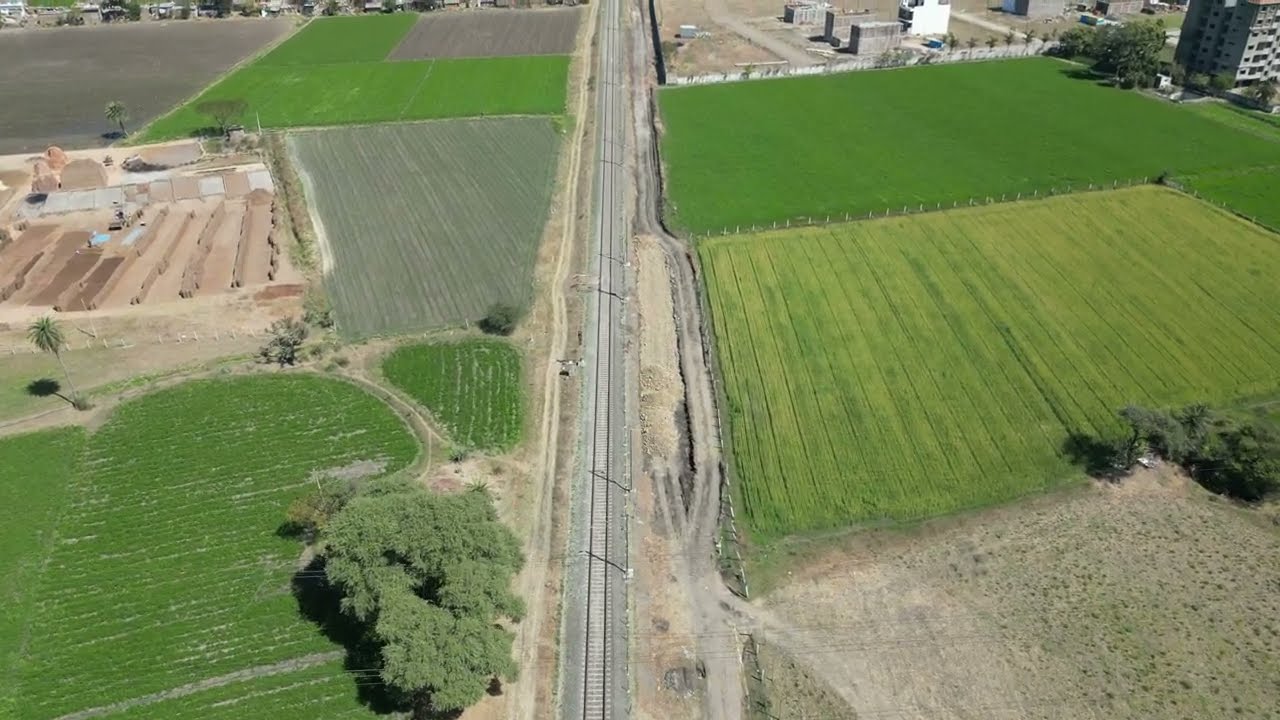This detailed, color, drone photograph in landscape orientation captures a high-altitude view of lush farmland bisected by a central railroad. To the left of the rail tracks, there are various patches of cultivated land, including lush green pastures and some fallow fields awaiting cultivation. A notably large tree is situated in the lower left-hand corner. To the right of the tracks, the landscape similarly features a mix of well-tended green fields and a couple of rougher patches that have been plowed or left as dirt with piles of stone. A prominent, multi-story building, presumably a high-rise apartment, stands in the upper right-hand corner, accompanied by a few other buildings visible in the background. The image's composition highlights the contrast between the orderly, green lots and the linearity of the railroad that slices through this picturesque agricultural scene.